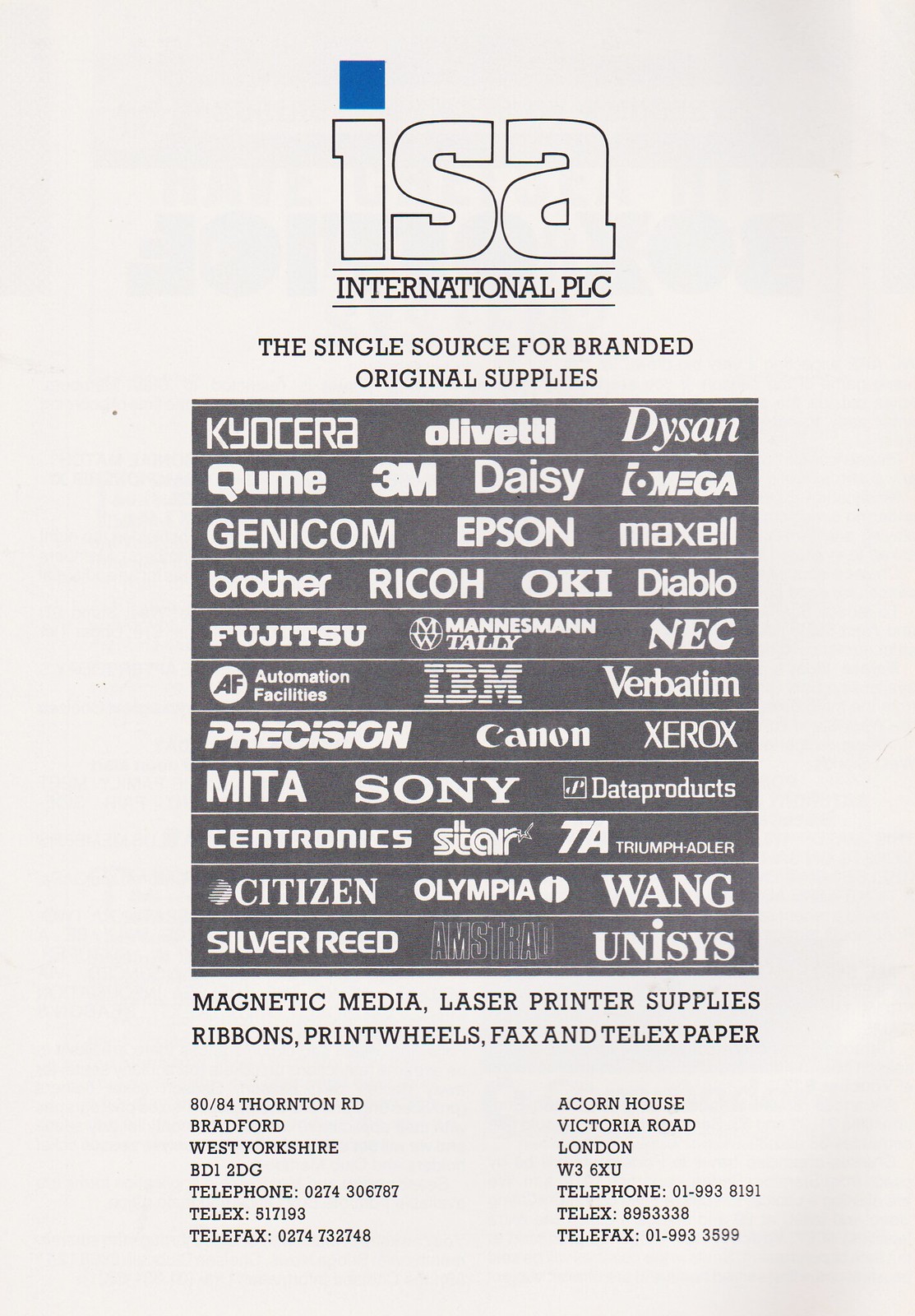The image is a vertical, rectangular, black-and-white cover of a trade publication, featuring a central theme of "ISA International PLC," emphasized as "the single source for branded original supplies." Positioned at the top is a small blue square, likely the dot for the letter "I" in "ISA." Below this header, a black text box appears, densely populated with various company logos and names, including notable brands such as Daisy, Epson, IBM, Canon, Xerox, Sony, Maxell, Fujitsu, Brother, Kyocera, Olivetti, and many others. This section indicates the brand diversity available. Following the logos is a listing that enumerates the types of supplies offered: magnetic media, laser printer supplies, ribbons, print wheels, fax, and telex paper. At the bottom, the publication provides the addresses, telephone numbers, and telefax numbers for ISA International PLC, arranged into two columns. The background of the poster has a grayish-white tone, reinforcing its professional and informational design.